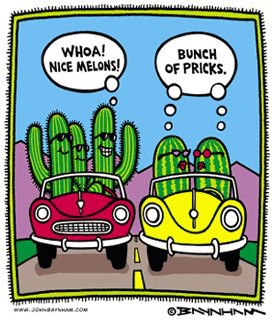This screenshot of a cartoon, with a slightly curved square dimension and small black hairs protruding from its yellow edges, captures a humorous scene on a flat road against a mountainous backdrop. The cartoon features a red convertible on the left, carrying three cactuses adorned with sunglasses. A text bubble above them reads, "Whoa, nice melons." Directly next to it, a yellow convertible drives alongside, occupied by two watermelons wearing glasses. Their text bubble responds with, "A bunch of pricks." The playful dialogue between the cactus and watermelon characters serves as a visual pun. The initials "B-N-Y-H-N-M" are subtly displayed in the bottom-right corner.